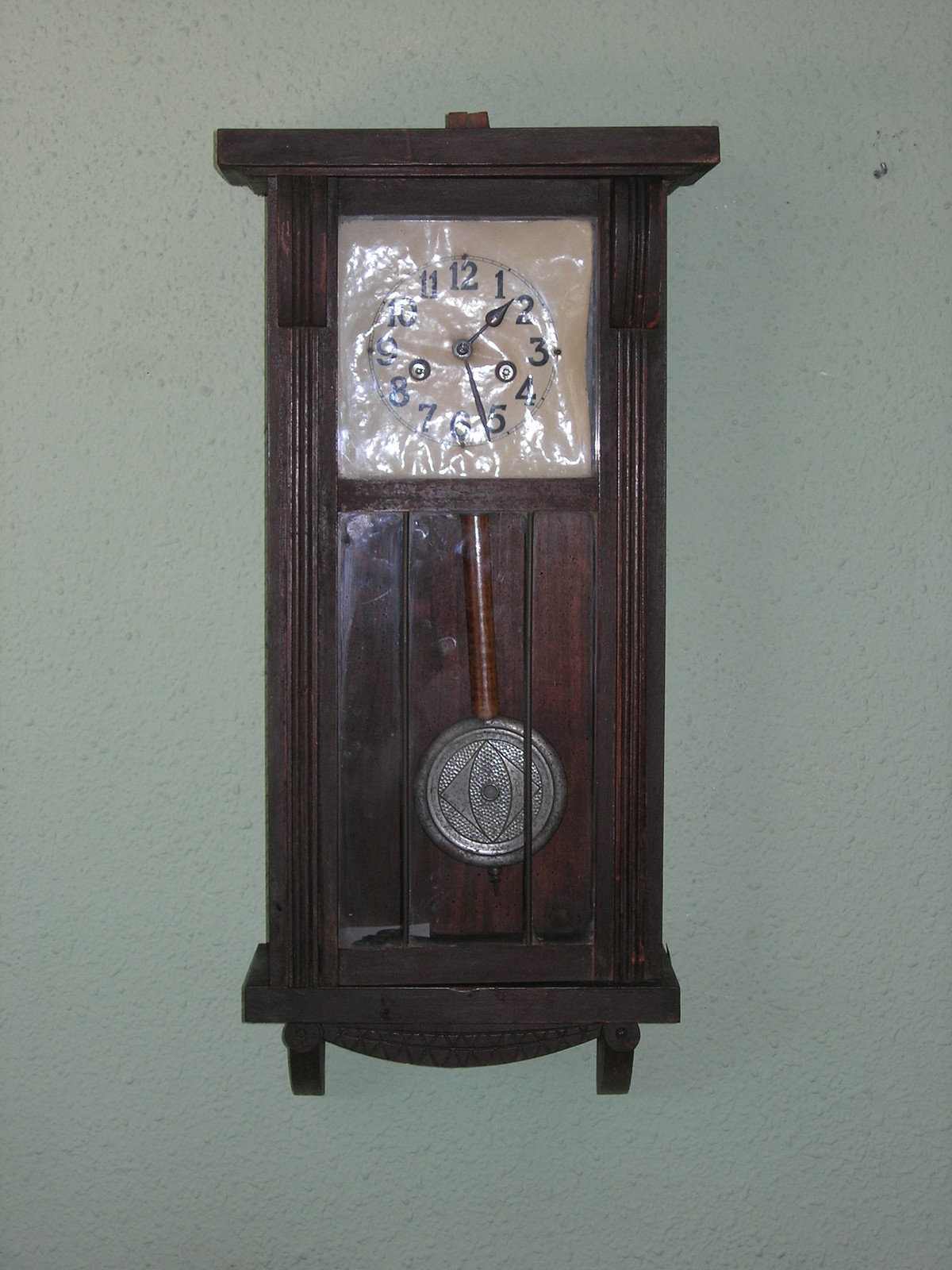This image depicts an old-fashioned, rectangular clock crafted from dark brown wood with a frame that extends slightly beyond its sides at both the top and bottom edges. The clock is mounted against a plain white, textured wall, often referred to as a popcorn wall. The clock has a prominent wooden ledge at the bottom and stands on small legs, adding to its vintage charm. Positioned above these legs, a wooden dome-like shape forms the base.

The upper part of the wooden frame houses the clock face, featuring a circular design set against a brown background that exceeds the size of the numerical area. The black numbers, indicating the hours, form a circle, with the number 12 at the top and 6 at the bottom. The black hour and minute hands mark the time just a bit after 1:25, protected by a clear, plastic-like glass cover.

Below the clock face, within a glass case, a swinging pendulum enhances its classic appeal. The pendulum, supported by a bronzy metal rod, is adorned with a silver emblem at its base, which showcases a triangular design reminiscent of an eye. Despite its antique essence, the clock bears signs of wear, including potential damage on the bottom left corner, hinting at its age and the stories it may hold.